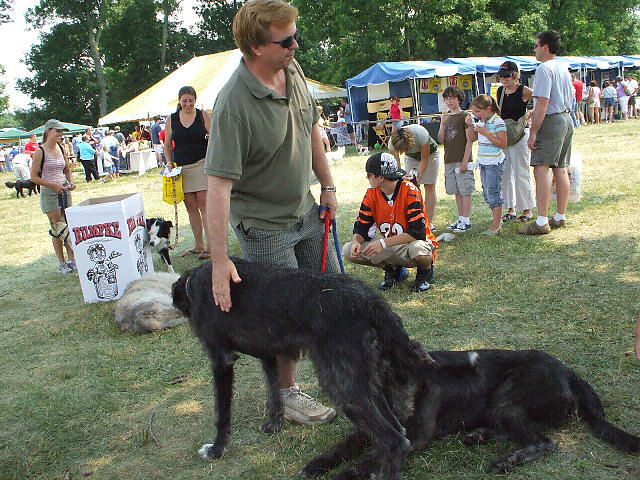This vivid photograph captures a bustling outdoor event set against a backdrop of partially cloudy skies and vibrant green, albeit slightly dry, grass. The scene is dominated by an array of tents—blue ones positioned to the right and a large white tent further back—indicating a lively fair or market setting. Closer to the foreground, a family, composed of a mother, father, and children enjoying ice cream, adds a touch of warmth and tenderness to the snapshot.

Front and center is a man, visibly enjoying the day, clad in a green shirt, shorts, and sunglasses, with dark blonde hair. He is affectionately petting one of two black dogs; this medium-sized canine stands facing away while another similar black dog rests on the grass nearby. In the immediate vicinity, more dogs are seen: one lounging and one standing beside a white cardboard trash can, with another woman nearby holding a dog on a leash. She dons a tan skirt, a black tank top, and carries a yellow bag. Another woman, sporting a hat, is also visible with a leashed dog behind the trash can.

The atmosphere buzzes with activity from patrons mingling and shopping, families enjoying the ambience, and a plethora of dogs scattered throughout. Trees stand tall in the distance, framing the event under a bright sky where the sun glistens, casting reflections on the ground.